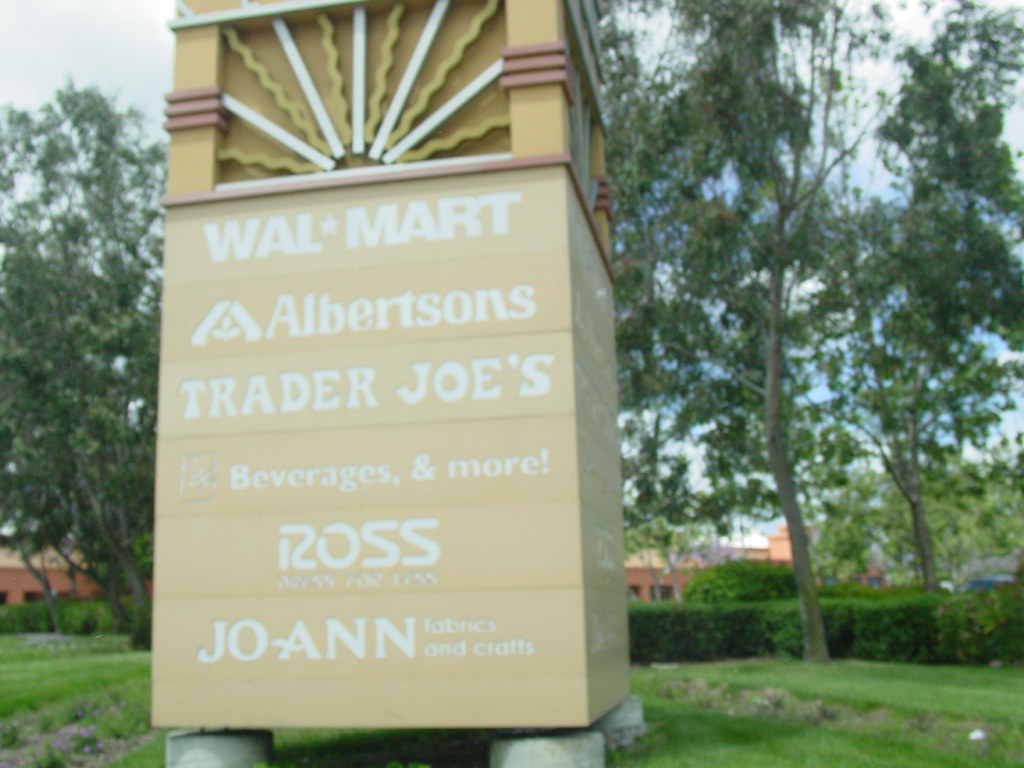The image depicts a partially viewed entrance sign to a shopping center. The sign, which is a large tanned square structure, is mounted on four round concrete blocks positioned towards the bottom left of the structure. Extending from these concrete blocks, two metal bars rise upwards, further supporting the bottom of the sign. 

At the top of the structure, a sunburst motif is prominently displayed. This motif is set within a carved-out rectangle and features white-painted wooden pieces arranged in a sunburst pattern, with yellow-painted squiggly wooden pieces forming a backdrop.

The sign lists a series of store names, all written in white. At the top is "Walmart," followed by "Albertsons," then "Trader Joe's," "Beverages Amore," "Ross Dress for Less," and finally "Joanne Fabrics." The right side of the sign indicates that these store names repeat.